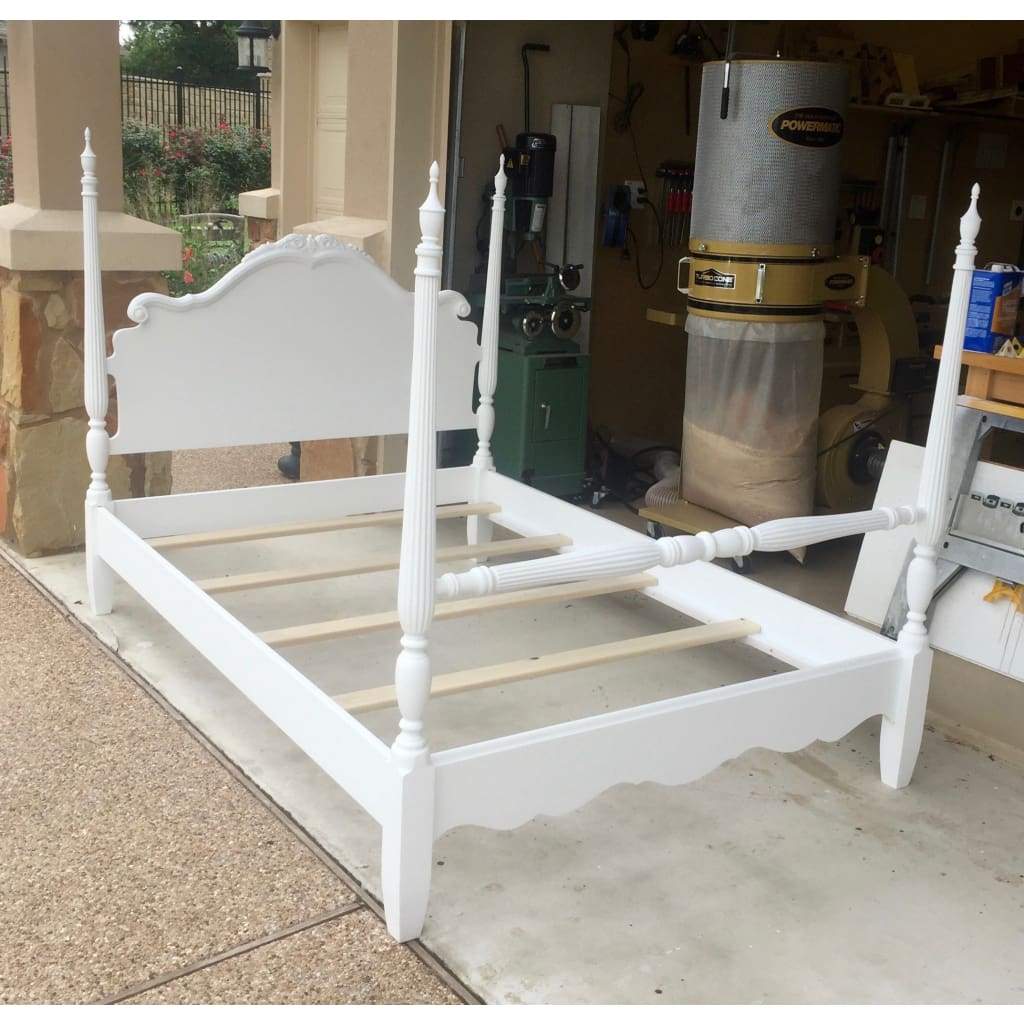In this exterior daylight photo, we see a detailed white wooden bed frame positioned in front of an open garage door. The bed frame, designed in an ornate style with French curls on the headboard, stands out with its four tall posts adorned with finials, reaching approximately six feet in height. The solid white-painted structure, including its supporting horizontal slats, is devoid of a mattress. The concrete floor beneath the bed adds a contrasting base to the pristine frame. The background reveals a glimpse into a woodworker’s shop within a garage, filled with woodworking tools and machinery, such as a dust collector and a drill press. Additionally, a water heater and various miscellaneous items are visible, emphasizing the garage setting. The meticulous craftsmanship and equipment suggest a dedicated workshop environment.